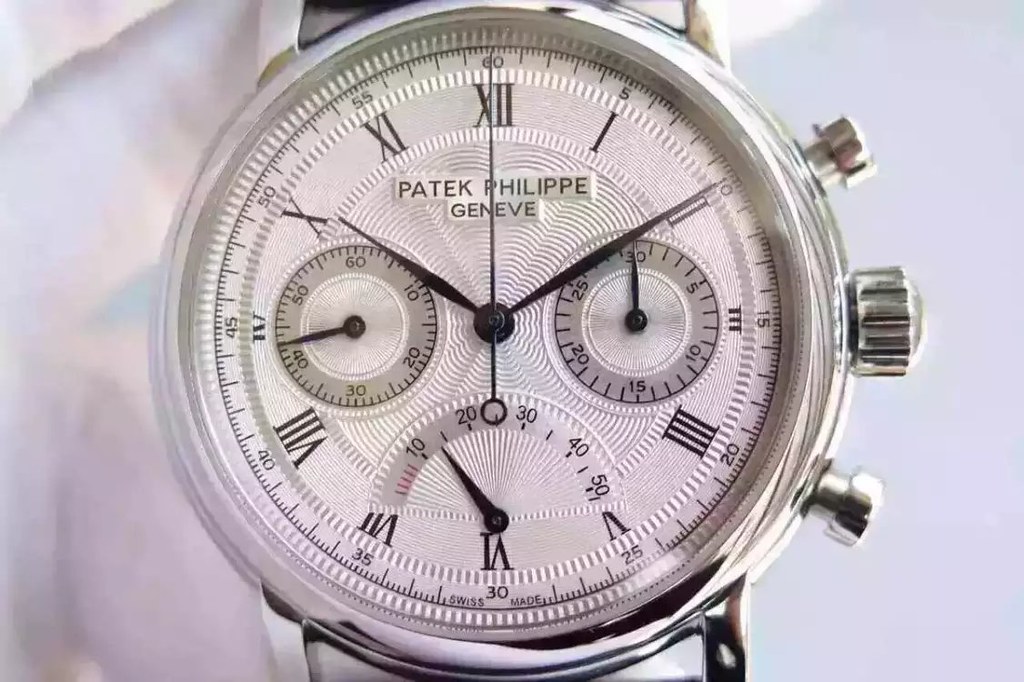This detailed photograph features a luxurious Patek Philippe Genève wristwatch against a smooth, white fabric background, resembling silk or fine linen. The watch's elegant face is encased in a silver-colored metal bezel, adorned with three distinct crowns on the right side for adjustments. The dial is predominantly white, showcasing a sophisticated blend of Roman numerals (I through XII) and regular numerals in increments of five from 5 to 60, with minute-marking lines between each numeral. Below the XII marker, the watch proudly displays the "Patek Philippe Genève" inscription. The dial also features two smaller sub-dials and a semi-circular sub-dial with detailed calibrations; one sub-dial measures up to 30, another up to 60, and the semi-circular dial ranges from 10 to 50. The bottom of the watch face is marked with "Swiss made," and the main hands of the watch are indicating the time 10:10.